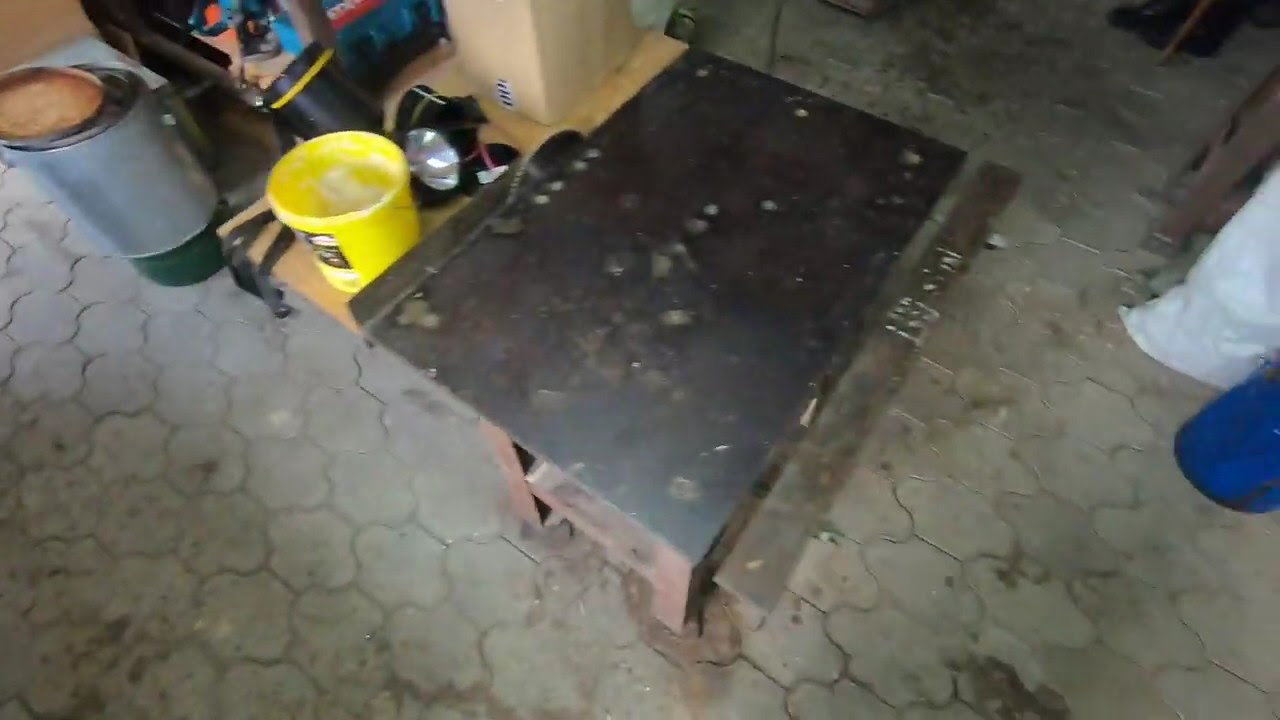This image captures a cluttered, somewhat blurry workshop scene with a concrete floor. Central to the image is a weathered workbench featuring a black, metallic surface and brown wooden supports, suggestive of an old, rusty appearance. The surface of the workbench looks dirty and worn, reflecting its frequent use. Directly behind the workbench, a bright yellow bucket stands out, accompanied by a gray, cylindrical metal container that sits on the ground. To the left of the workbench, you can find a wooden table bearing a headlamp. Scattered around, there are various items, including white and royal blue objects that resemble tarps or rolled-up materials. Additionally, a white piece, possibly cloth or plastic, rests on the right side of the image. The area is quite dirty, with the floor made up of different pieces of concrete, contributing to a chaotic and rugged atmosphere in what seems to be a highly functional, albeit unkempt, workspace.